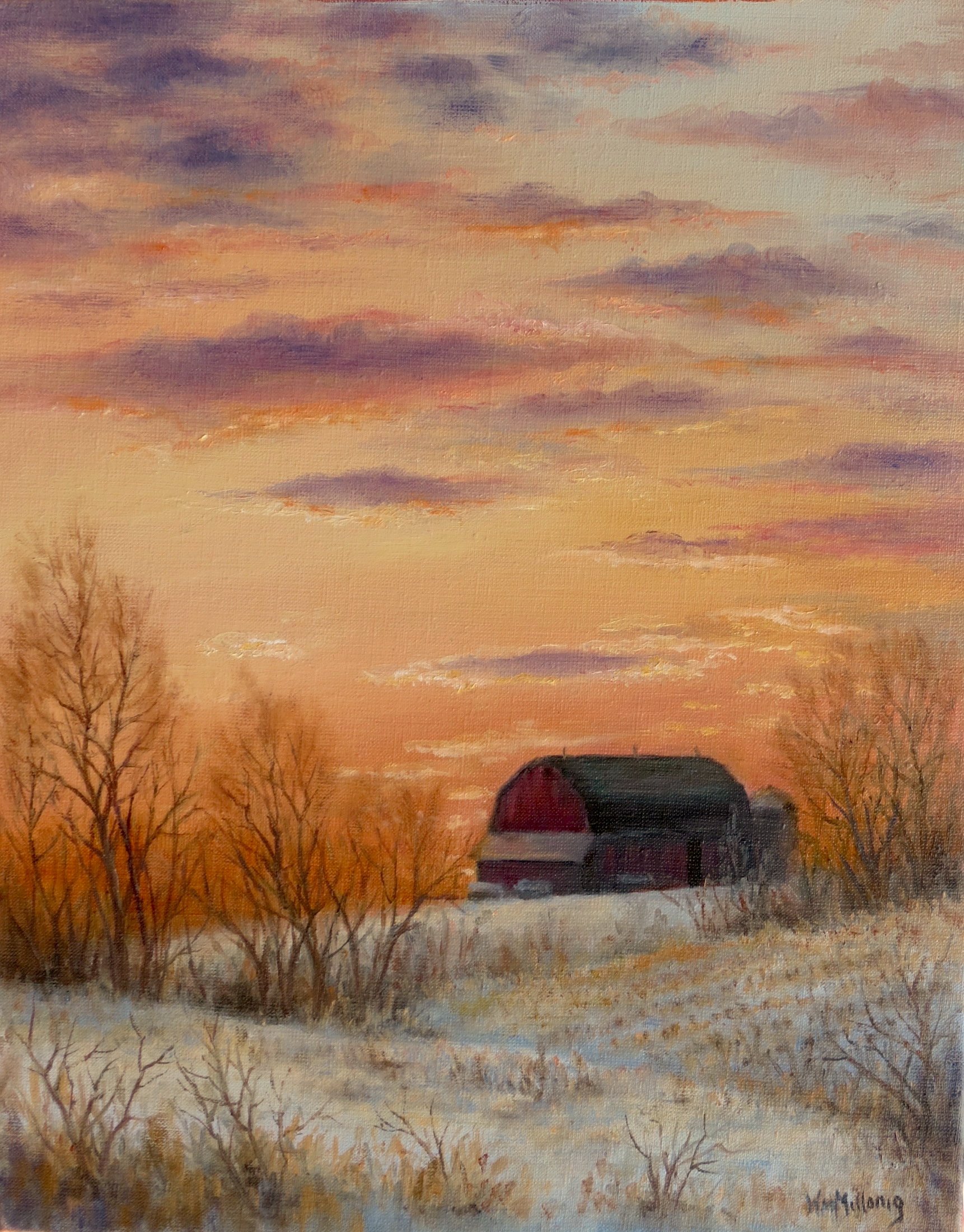This painting, a captivating winter landscape, showcases a traditional Dutch-style red barn with a black roof lightly dusted with snow. Positioned towards the background, the barn is accompanied by a grain silo behind it, reinforcing its role in a farm setting. The foreground features barren trees with no leaves and snow-covered ground, indicating a cold, wintry scene. A field extends to the right of the image, partially covered by scrub brush. The sky is a mesmerizing blend of sunrise or sunset hues, with orange, yellow, and purple clouds illuminating the scene. The artist's signature, though difficult to decipher, is visible in black paint at the bottom right of the frame.